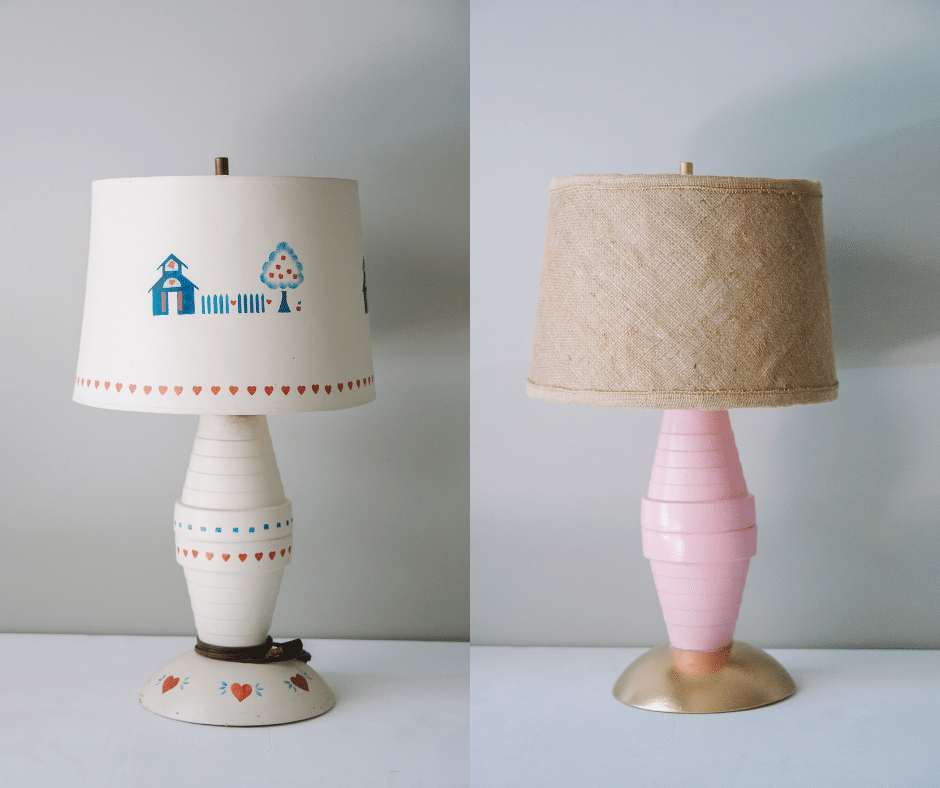The image showcases two creatively crafted lamps positioned side-by-side against a grayish-white wall with a white surface beneath them. The lamp on the left features a white, tube-like base that looks like two flower pots joined top-to-top, with decorative motifs. Orange-red hearts with blue accents adorn the base, complemented by a whimsical lampshade. The lampshade itself is white, decorated with charming scenes—a blue house with a heart and picket fence, a blue tree speckled with red apples, and a bottom border of red hearts. A white cord is neatly wrapped around the base.

On the right, the lamp offers a contrasting, uncluttered design. Its base consists of a gold-colored inverted bowl with a pink section above it, maintaining a minimalistic aesthetic. The lampshade is made of a buff-colored, natural woven material. This lamp, much like the one on the left, sits on a white surface under similar shadowy lighting, highlighting the comparison between the ornate and the simple elegance of these two lamps.